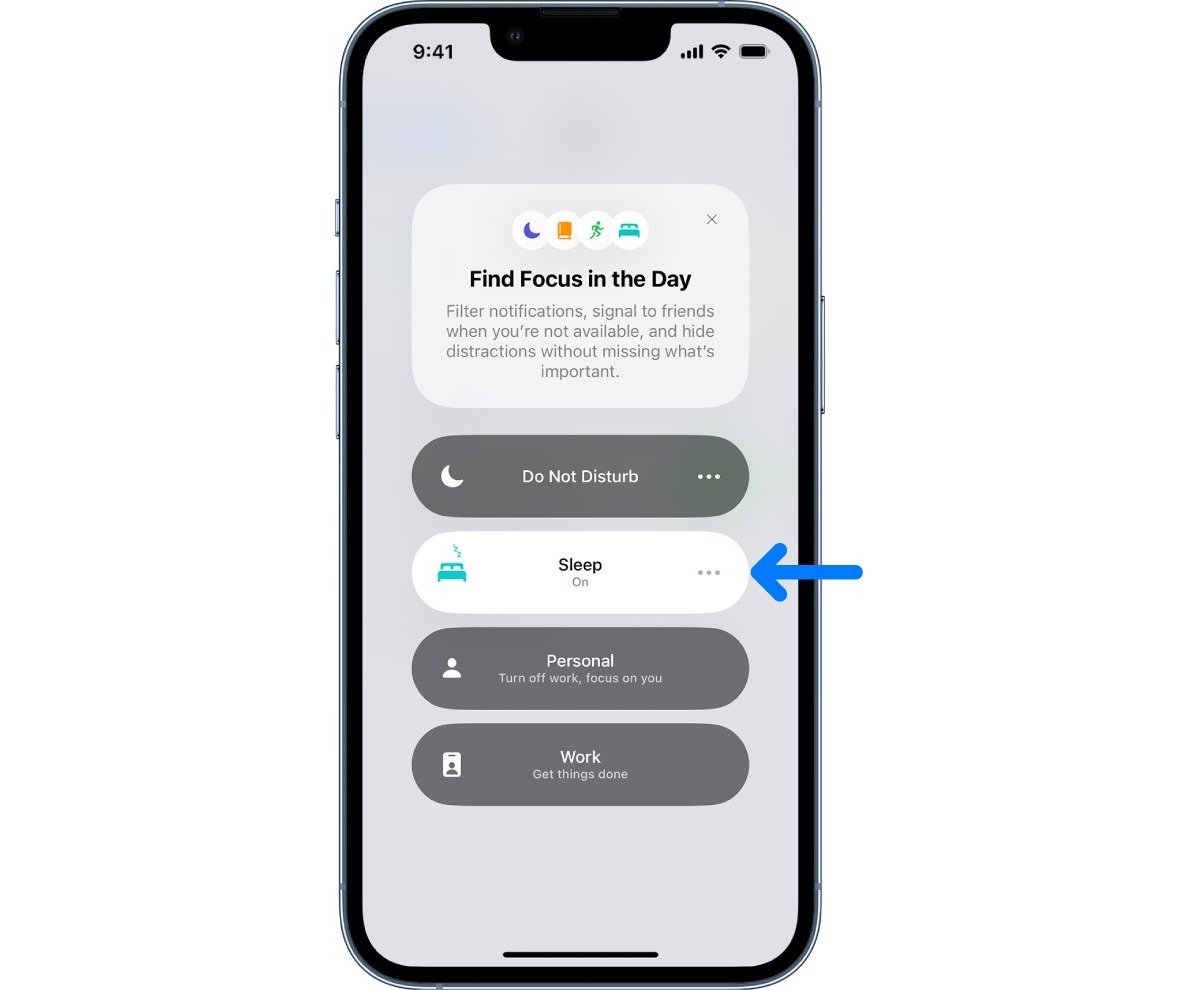This image is a smartphone screenshot taken at 9:41, with a full battery and a connected Wi-Fi signal visible at the top of the screen. In the center of the screen, there are three symbols: a horizontal moon indicating "Do Not Disturb," an icon resembling a bed, and another icon that is difficult to identify but mentioned as related to the main function. A notification box in the middle of the screen contains text advising the user to "Find focus in the day" by filtering notifications, signaling to friends when they are unavailable, and hiding distractions without missing important updates.

Below this notification box are options related to different focus modes. The first option, marked with a moon and three dots, corresponds to "Do Not Disturb." The second option, highlighted by an arrow in the screenshot, shows a bed icon and is labeled "Sleep." It states "Sleep on," and implies a mode focused on resting. Below the bed icon, there are two more categories: "Personal," depicted by a person's icon with a message to "Turn off work. Focus on you," and "Work," illustrated by an ID tag icon, urging the user to "Get things done."